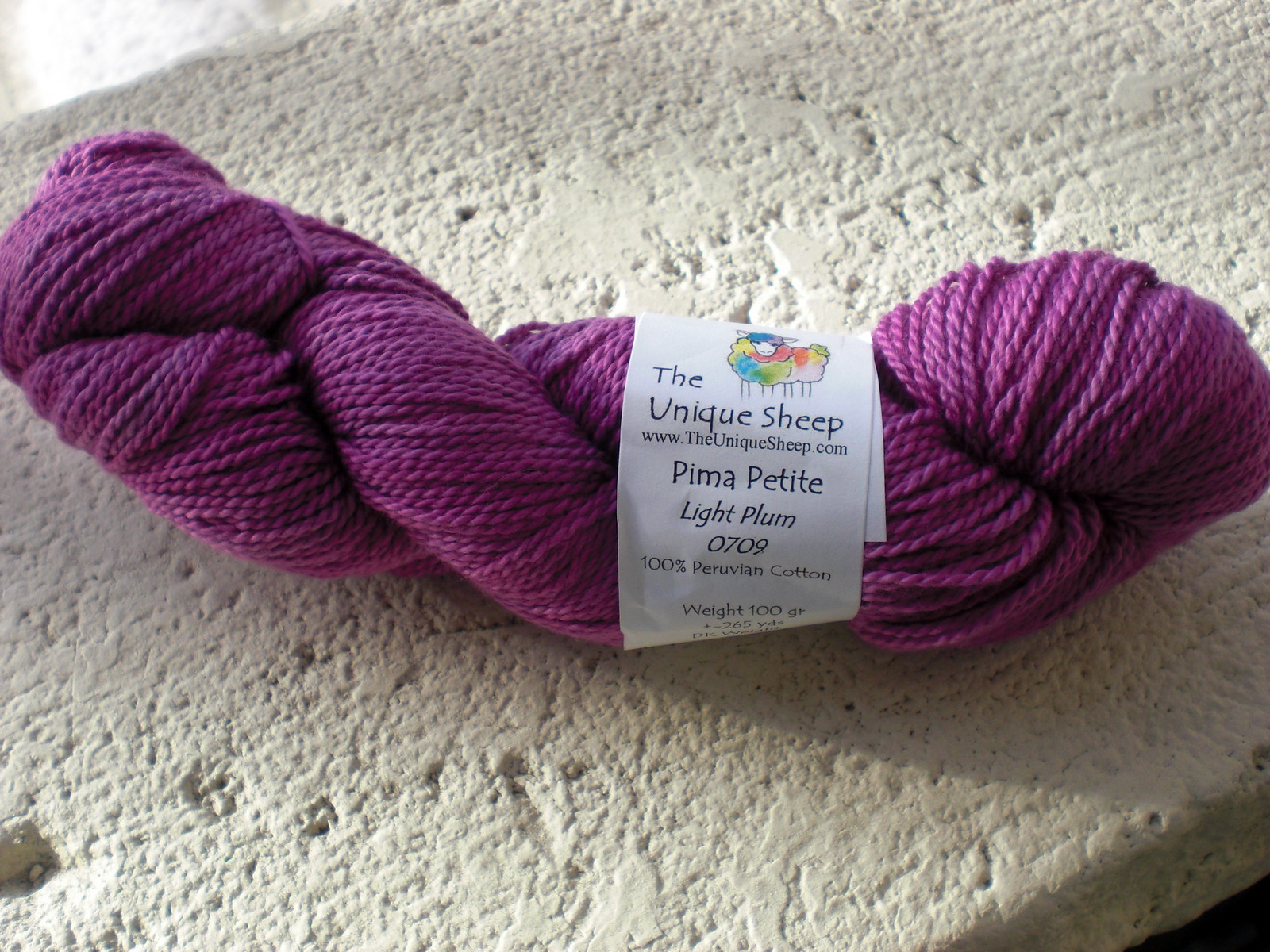The image is a close-up of a fresh, unused, dark purple ball of yarn, specifically labeled as "The Unique Sheep" Pima Petite Light Plum 0709, weighing 100 grams and 264 yards in length. The yarn is a two-strand twist made up of numerous fine strands, creating a thick and well-twisted texture. It is encased in a white wrapper featuring a multi-colored sheep and the website www.theuniquesheep.com. The ball of yarn rests on a white, porous concrete shelf that has numerous small holes, indicating its rough texture. The photograph, taken during the day, captures the sun shining on the yarn, enhancing the vibrant color and texture of both the yarn and the surface it sits on, highlighting the details of the setting which is indoors.